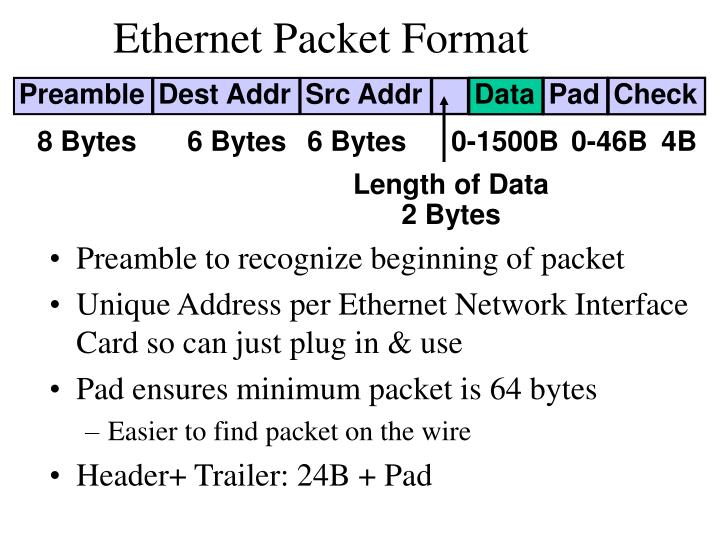The image is a detailed text-based chart titled "Ethernet Packet Format." The format is outlined within a rectangular purple box, subdivided by various segments with their respective labels and byte sizes. Each segment is color-coded, with the 'Data' segment distinctly highlighted in green. The segments read in sequence: "Preamble," "Destination Address," "Source Address," "Data," "Pad," and "Check," indicating their roles and sizes. Below the primary labels, specific byte sizes are noted: "8 bytes" for the Preamble, "6 bytes" each for the Destination and Source Addresses, "0 to 1500 bytes" for Data, "0 to 46 bytes" for Pad, and "4 bytes" for Check. Additional text elucidates their functions: the Preamble helps recognize the packet's beginning, destination and source addresses are unique per Ethernet network interface card, the Pad ensures the minimum packet size is 64 bytes, and the total header and trailer length is 24 bytes plus the Pad. This chart provides comprehensive information essential for understanding Ethernet packet structure.